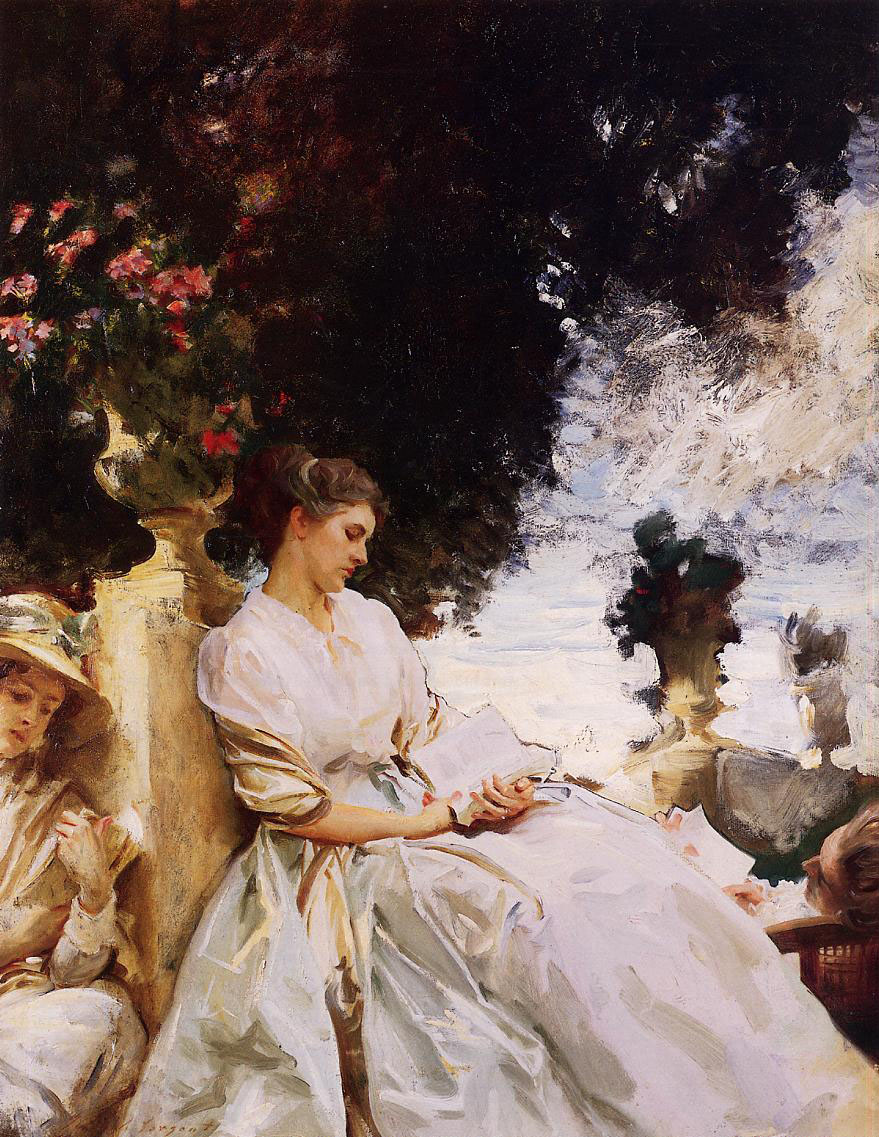An oil painting depicts a tranquil outdoor scene featuring two women. In the foreground, a woman with dark brown hair tied back into a ponytail sits and leans against a yellow stone wall. She wears a voluminous, wide, cream-colored dress with semi-transparent white fabric at the top, revealing hints of her skin. A gold-colored scarf drapes around her shoulders and arms. Her gaze is directed downward at an open book resting on her lap, one hand holding the book up while a finger from her other hand touches a page.

Next to her, partially visible, is another woman who also wears a voluminous cream dress, accented by a tan hat adorned with a green flower. She holds a book with one hand, looking down at its pages, her head positioned near the first woman's shoulder.

Above and behind them, a large, almost black tree with red accents looms against the sky, which contains a few wispy clouds. A stone pillar stands behind the seated woman, topped with a golden flower pot filled with green leaves and red flowers. To the right, a partial view of another person with backward-combed brown hair leans against a chair, their face partially obscured. The scene is bathed in a palette that includes yellow stone, green foliage, red flowers, and the soft creams of the women's dresses, contributing to the leisurely and serene atmosphere of the painting.